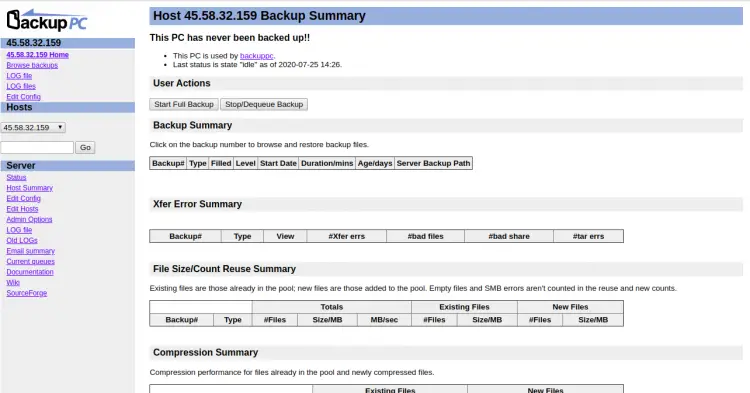Here is a detailed and cleaned-up caption for the described image:

---

The image captures a screenshot of a computer screen displaying a backup program interface called "Backup PC." The logo for "Backup" cleverly incorporates the letter 'B' shaped like a floppy disk, followed by "A-C-K-U-P". "PC" is written in capital letters. An arrow pointing left is located at the upper part of the "Backup" logo. 

On the far left of the screen, there is a column featuring what appears to be a router or IP address: 45.58.32.159. This section includes several menu buttons, beginning with "Home," followed by "Browse," "Backups," "Log File," "Log Files," "Edit Config," and "Hosts." Below these buttons, the column features two vertical rectangular input boxes accompanied by a "Go" button.

Further down, there is a list of servers, each with its own status button, followed by menu options like "Host Summary," "Edit Config," "Edit Host," "Administration Options," "Log File," "Old Logs," "Email Summary," "Current Menus," "Documentation," and a link to "SourceForge."

To the right of this column is the main screen area, which provides detailed information about the backup status for the host with the IP address 45.58.32.159. At the top is a blue title bar that reads "Backup Summary." The main content indicates that the PC has never been backed up, showing various summaries, including "User Action," "Backup Summary," "X for Error Summary," "File Size/Count," "Reuse Summary," and "Compression Summary."

---

This detailed caption offers a comprehensive textual description of the image, ensuring clarity and coherence.